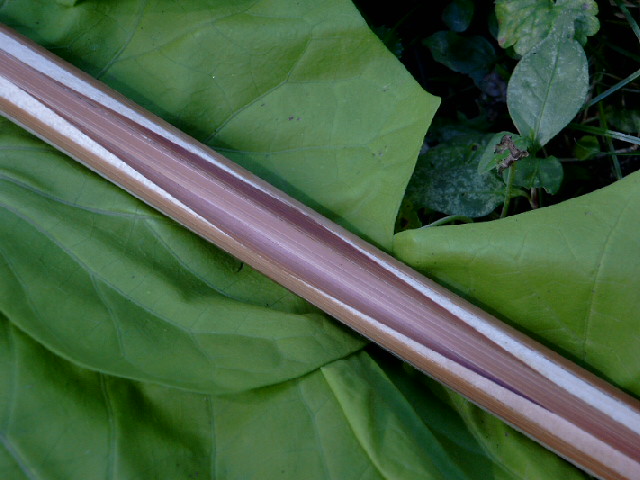In the image, a striking contrast is created with a fibrous, pinkish-purple object, resembling the handle of a pen, resting on lush, vibrant green leaves. This close-up reveals the intricate details of the leaves which vary in size, some large and others smaller, all appearing very healthy, moist, and intact with slight wrinkles indicating their hydration. The central object, likely a cut stem, shows a fibrous, dark brown exterior with hints of white trim where it has been freshly split open, adding a textural depth to the image. The scene is set against a backdrop of grass and other plants, some with signs of aging or insect damage. Additionally, scattered petals and possibly a blue flower can be faintly discerned, adding subtle complexity and richness to the composition.